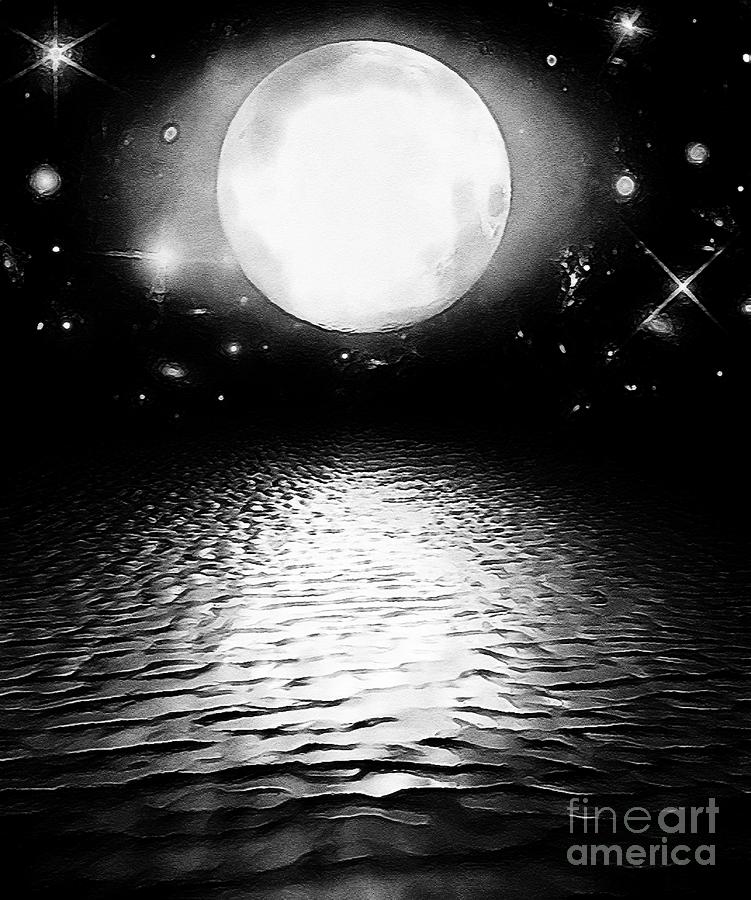This is an artistic depiction in black and white, likely a painting or charcoal drawing, featuring a luminous moon positioned about one-third from the top center of the image. The enchanting night sky, providing the backdrop, is filled with deliberately painted stars, some with intricate rays emanating from them. Surrounding the moon is a striking halo of radiated light and various patterns, including swirls and tiny crosses, suggesting distant star systems or planets. The foreground appears to illustrate a textured, rippled surface that might be water or a slick pattern of rock, accentuated by the moon’s reflection. Despite its ambiguity, this surface features a pronounced diffuse highlight, adding depth and intrigue to the scene. The piece emanates a dark, mysterious ambiance with the phrase "Fine Art America" inscribed at the bottom right.